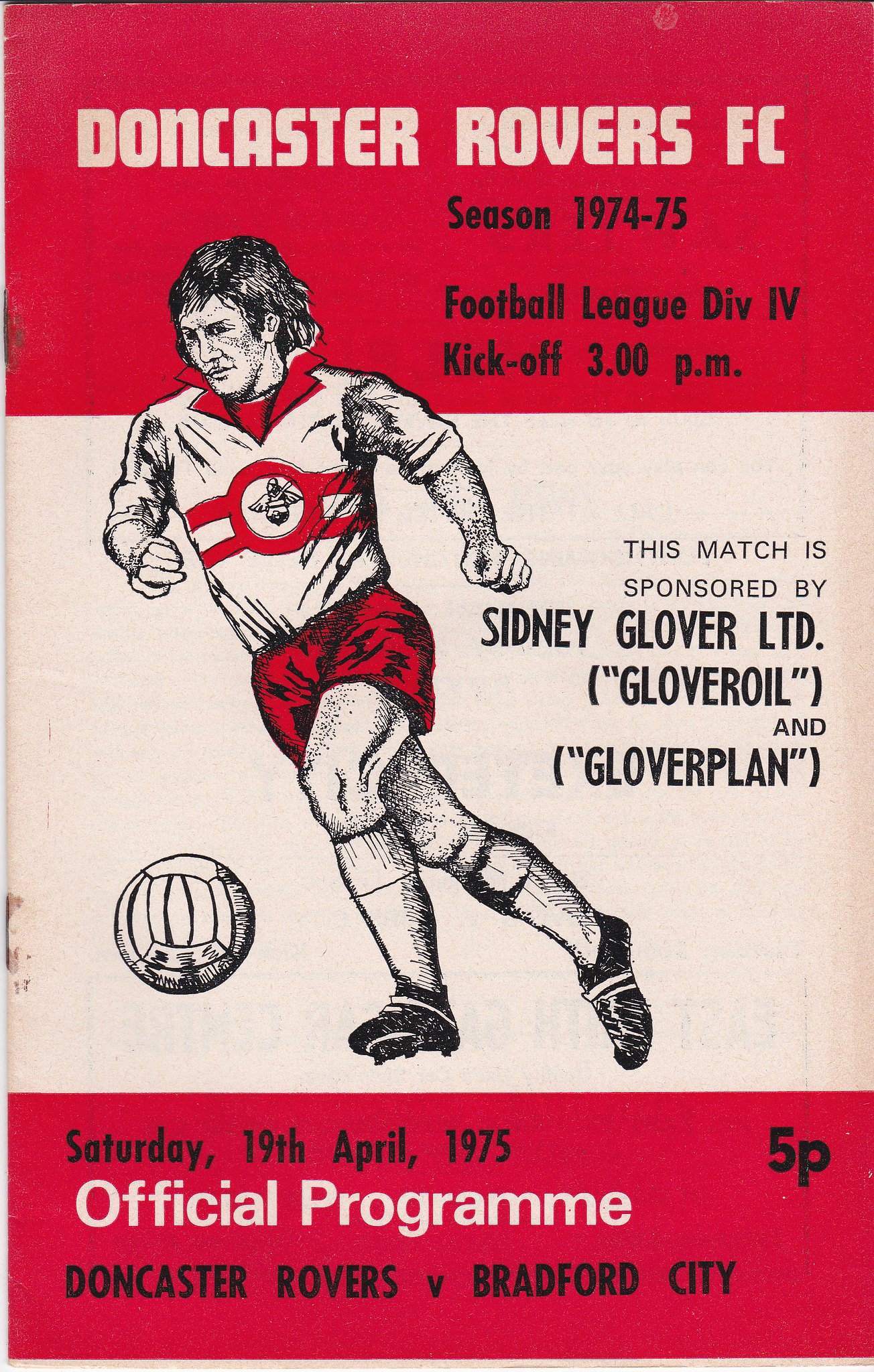The image is a reproduction of the official program for the Doncaster Rovers Football Club match against Bradford City, dating from the 1974-75 season. The program, priced at five pence, features a red and white color scheme. At the top, a red rectangle with white text reads "Doncaster Rovers FC," followed by "Season 1974-75, Football League Div. IV, kickoff 3 p.m." in black text. Below this, a large white rectangle contains an illustration of a football player kicking a soccer ball. The player, with black longer hair, is depicted in a red and white uniform comprising a white polo shirt with a red collar and decorative stripe, red shorts, white socks, and black cleats. The central figure and ball are well-positioned, enhancing the visual appeal. Additionally, the program notes that the match is sponsored by Sidney Glover Limited, Glover Oil, and Glover Plan. The bottom part of the program has another red band with white and black text stating "Saturday, 19th April 1975, official program, Doncaster Rovers vs. Bradford City," with the price listed as "5p."